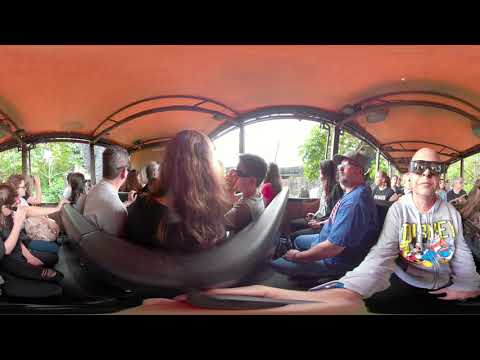The image depicts a lively scene featuring a group of people in what appears to be an outdoor adventure ride or a themed bus tour, possibly at a place like Walt Disney World. The photograph is framed by thick black borders both at the top and bottom. In the background, an orange, curved ceiling creates arches through which lush greenery is visible, suggesting an outdoor environment.

The scene is bustling with around two dozen individuals, seated and facing in various directions. Central to the image is a rounded gray booth where three people are particularly noticeable. On the left of the booth, a man with grayish hair in a white shirt faces slightly to the right. In the middle, a woman with long brown hair faces away, while to the right, a man with short dark hair and sunglasses gazes to the left.

To the right of this group, another man in a blue shirt and hat also faces left. Adjacent to him is a striking figure: an older woman wearing dark sunglasses and a distinctive long-sleeved shirt with an unreadable text and Mickey Mouse and Pluto illustrations, suggesting a Disney-themed outing. Her right arm extends forward, with the hand appearing distorted at the bottom of the image, likely holding a camera that took the picture.

The overall impression is that of a warm, overcast day, given the visible ceiling and attire of the people. While the exact setting remains ambiguous—be it a themed ride, a bus, or a patio extension of a restaurant—the engaging expressions and varied orientations of the individuals capture a moment of shared excitement and curiosity.